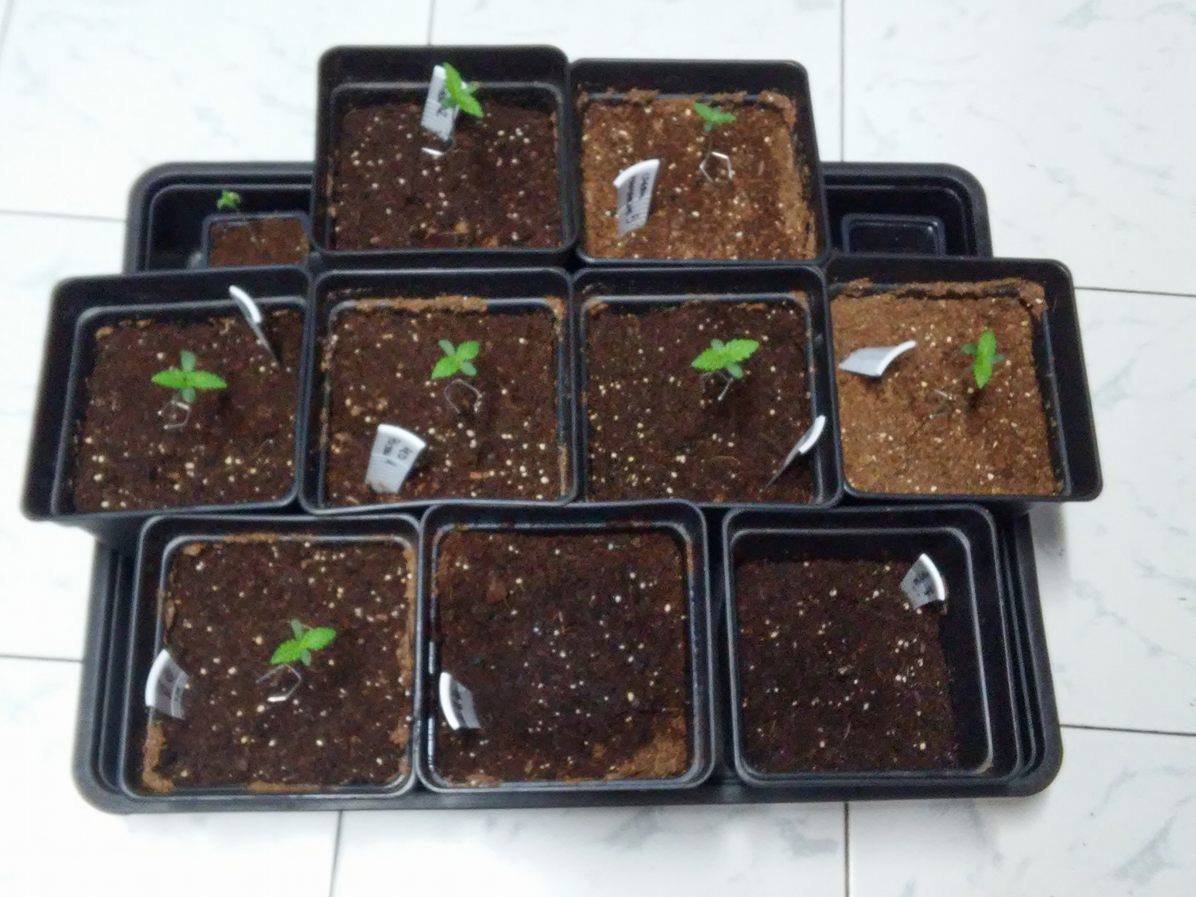The image captures a bright but blurry photograph of early seedling plants arranged in black, likely plastic, square plant pots. The scene is set against a background of white marble tile flooring, possibly in a kitchen. The pots are organized in multiple rows stacked on top of each other within a larger black container; visible are three rows with two pots in the top row, four in the middle, and three in the bottom row. Each pot contains dark soil with occasional white specks, and most pots, except for two in the bottom right, have tiny green seedlings emerging with leaves resembling mint—dark green with oblong shapes and jagged edges. A few pots appear to have drier soil, particularly the top right and the last middle-right pot. Unreadable tags are present in the containers, hinting at the organized planting effort.